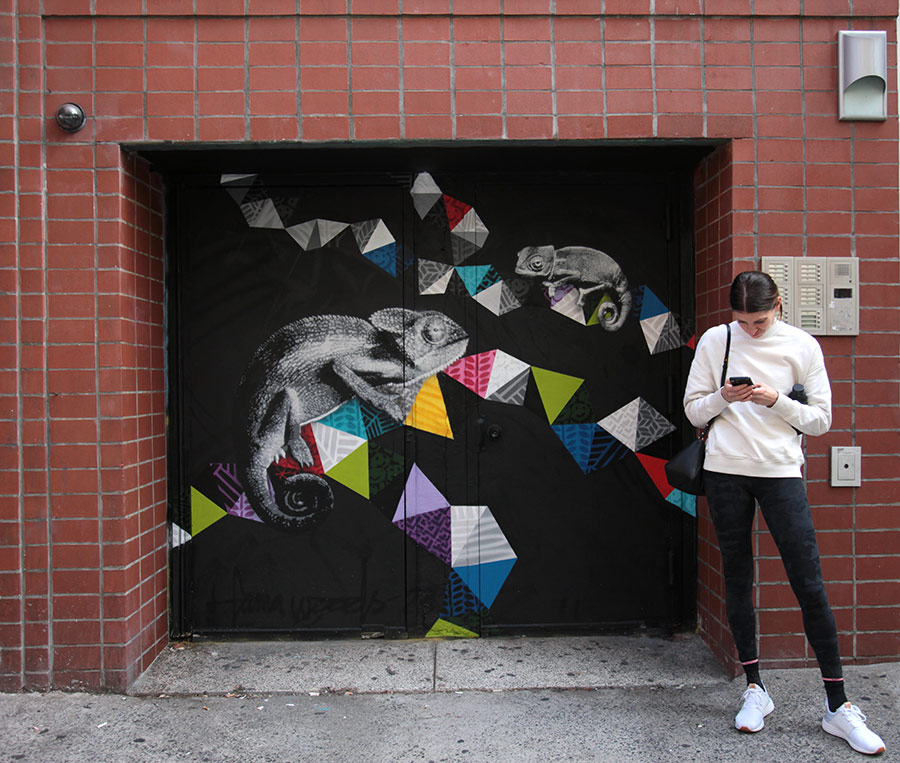In this photograph, a woman stands on a sidewalk against a backdrop of a red brick building. Positioned on the right side of the frame, she’s attired in a white long-sleeve shirt, black pants or leggings, and white shoes. She holds a black purse on her right arm and is engrossed in her black cell phone, which she clutches with both hands. Directly behind her, there is a black door adorned with silver chameleons—mistaken for iguanas by one observer—and vibrant triangles in colors such as purple, blue, green, yellow, and white, which either decorate the areas around the chameleons or serve as their perches. Above her head, attached to the brick wall, is a silver rectangular box with buttons, possibly functioning as a buzzer to gain access to the building's black doors.